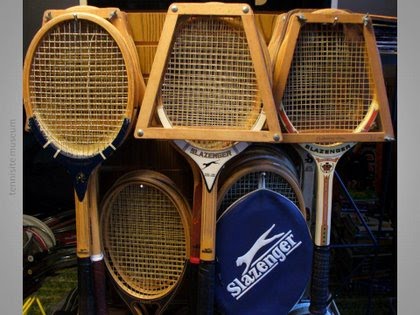This image showcases a collection of wooden tennis rackets arranged in rows. At the top, a row of three wooden tennis rackets is visible, with another row directly behind them. On the left, there is an oval-shaped racket framed by a matching oval wooden frame. In the middle, there is a tennis racket with a white edge at the bottom, and in front of it, a wooden trapezoid frame. Similarly, on the right, another tennis racket with a white border is framed by a trapezoid wooden shape. The brand name "Slazenger" is visible on these rackets, noted for its distinctive white lettering. At the bottom, there is another row of tennis rackets, with two prominently displayed and more behind them. One of these rackets is partially covered by a blue cover with white text, also bearing the "Slazenger" name and an outline of a cheetah above the text. The background of the image appears dark, making the wooden textures and brand details stand out.